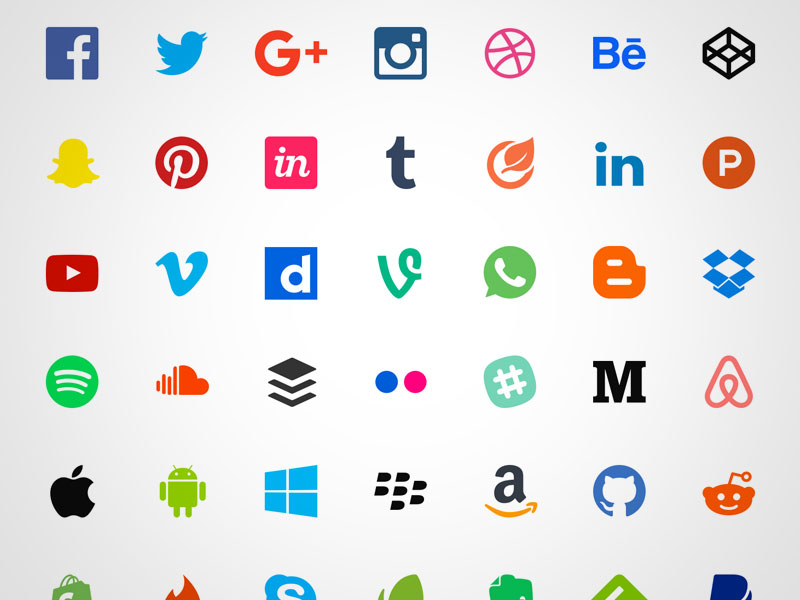This photograph captures an array of recognizable tech company logos arranged in a structured grid. There are six and a half rows and seven columns showcasing a variety of symbols, with some partially cut off at the edges. The logos include Facebook, Twitter, Google+, a camera icon (possibly Snapchat), and a basketball. Additionally, there’s BE, a black square (possibly Instagram), Pinterest, an INT logo, a leaf symbol, the LinkedIn "IN", and an orange circle with a "P". The photograph also features YouTube, Vimeo, a "D" (possibly Dropbox), a green phone icon (maybe WhatsApp), a red-and-white striped symbol, a cloud icon, contactless payment symbols, and an Amazon logo. There are also less recognizable logos, such as a pink and blue dot, a letter "M", and a tech-related robot image. Famous logos like Apple, Audible, Spotify, Microsoft, and Reddit are noticeable among others. The grid pattern is neatly organized, offering a panoramic view of several well-known and lesser-known tech and social media brands.